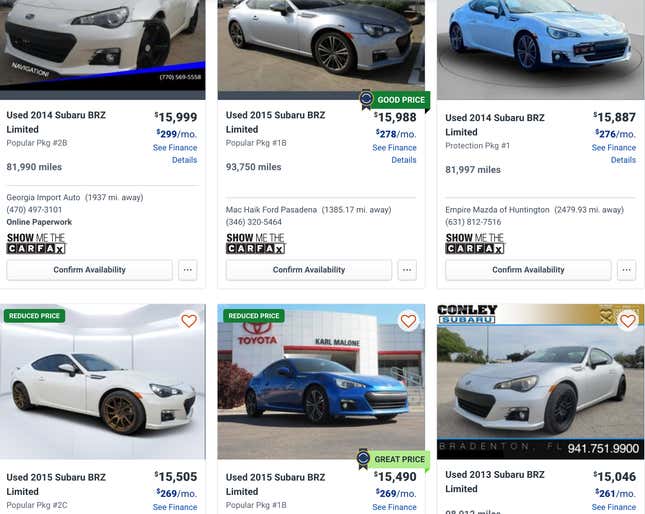A pre-owned 2014 Subaru BRZ Limited, priced at $15,999, is showcased in this image. The vehicle features a sleek white exterior complemented by a stylish black grille and black wheels, suggesting a sporty and sophisticated design. The car has accumulated 81,997 miles and offers a financing option of $269 per month. This particular model is well-regarded for its balance of performance and aesthetics, making it a popular choice among driving enthusiasts. The dealership provides this vehicle as part of their quality used car inventory, ensuring it has undergone thorough inspections to meet industry standards.